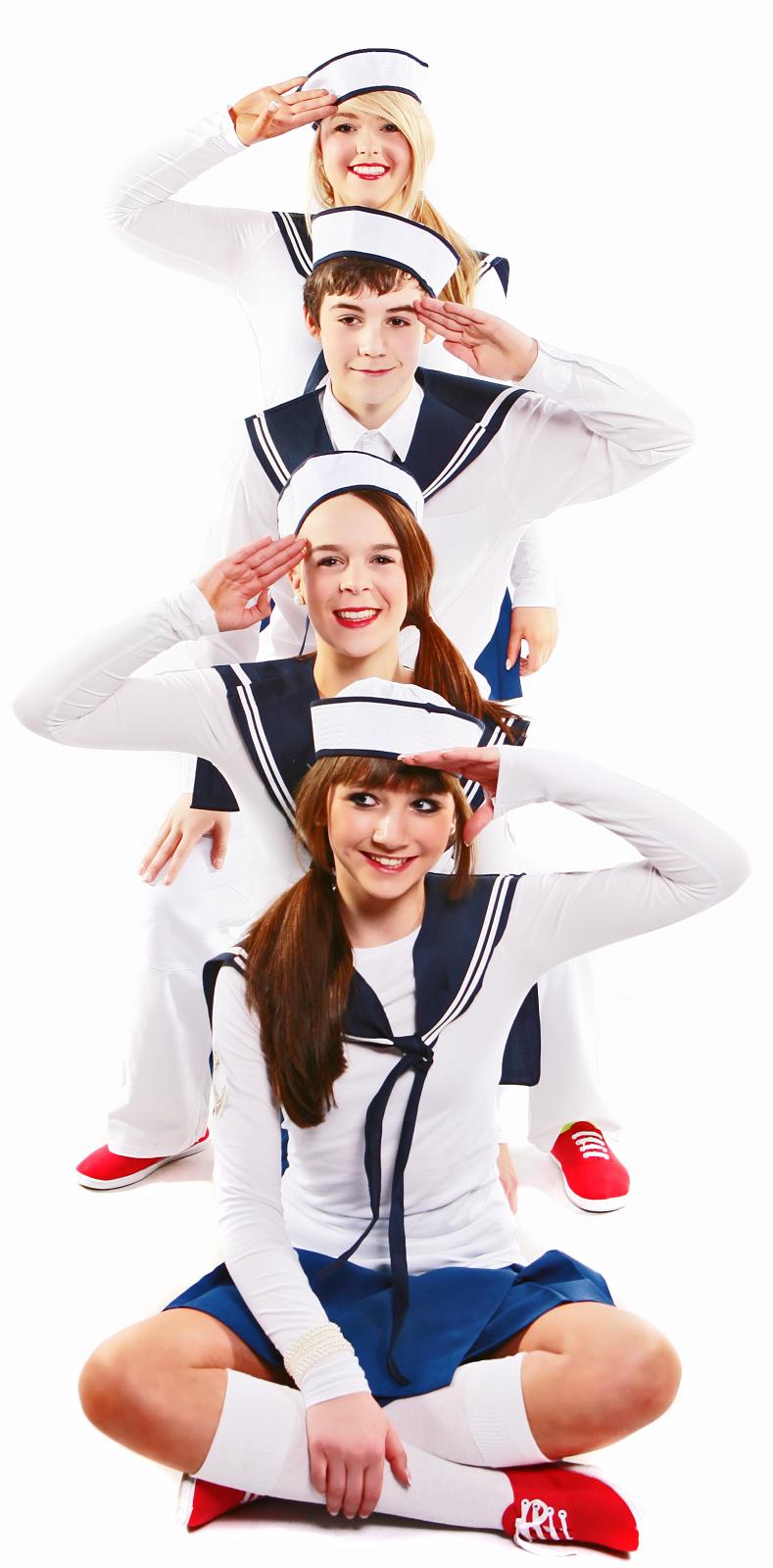In a studio photograph with a white background, four young individuals—three girls and one boy—are modeling novelty sailor outfits. They are arranged in a vertical line from front to back, with the front model sitting cross-legged, followed by two kneeling, and the final model standing. The front girl has long brown hair draped over her shoulder, a blue and white sailor hat, and a blue skirt paired with a white long-sleeve shirt featuring a blue sailor collar. She is saluting with her left hand while looking to the left, smiling. Behind her, another girl with dark hair is kneeling, also adorned in a blue and white sailor outfit with knee-high white socks and red shoes, saluting with her right hand and looking straight ahead. The boy, kneeling as well, is the third in line, donning white sailor pants—a nod to traditional bell-bottoms—and a blue and white sailor top. He is saluting with his left hand and looking off to the left, smiling. At the very back stands a blonde-haired girl with a sailor hat, saluting with her right hand, her hair partially covering one eye as she smiles brightly. Each model wears red sneakers, completing the coordinated ensemble of sailor outfits.